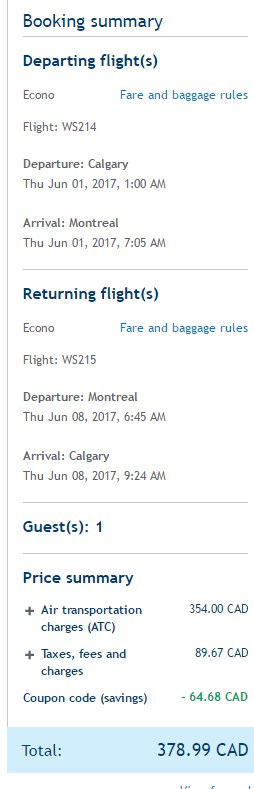This image is a long, narrow screenshot, presumably extracted from a digital booking summary, significantly exceeding the standard screen length. The document provides comprehensive flight details for a trip to Cano. It starts with a "Booking Summary" header in blue font, followed by the trip information organized in a typewriter-style black font.

Key details include:
- **Departing Flight**: 
  - **From**: Calgary
  - **To**: Montreal
  - **Date and Time**: Thursday, June 1st, 2017 at 1:00 AM
  - **Arrival**: Thursday, June 1st, 2017 at 7:05 AM

Additional clickable details like "Fare and Baggage Rules" are available. There is also a section for the returning flight information, passenger details, and cost breakdown. The cost summary, including air transportation fees, taxes, and any applied coupon savings, amounts to $378.99 CAD. The headers like "Booking Summary," "Departing Flight," and "Returning Flight," along with the price summary, are emphasized in blue and bold. The total cost is highlighted within a light blue box, adding a structured and professional touch akin to a meticulously crafted spreadsheet.

The image background is white, allowing the blue and black text to stand out clearly, giving it a clean and organized appearance.